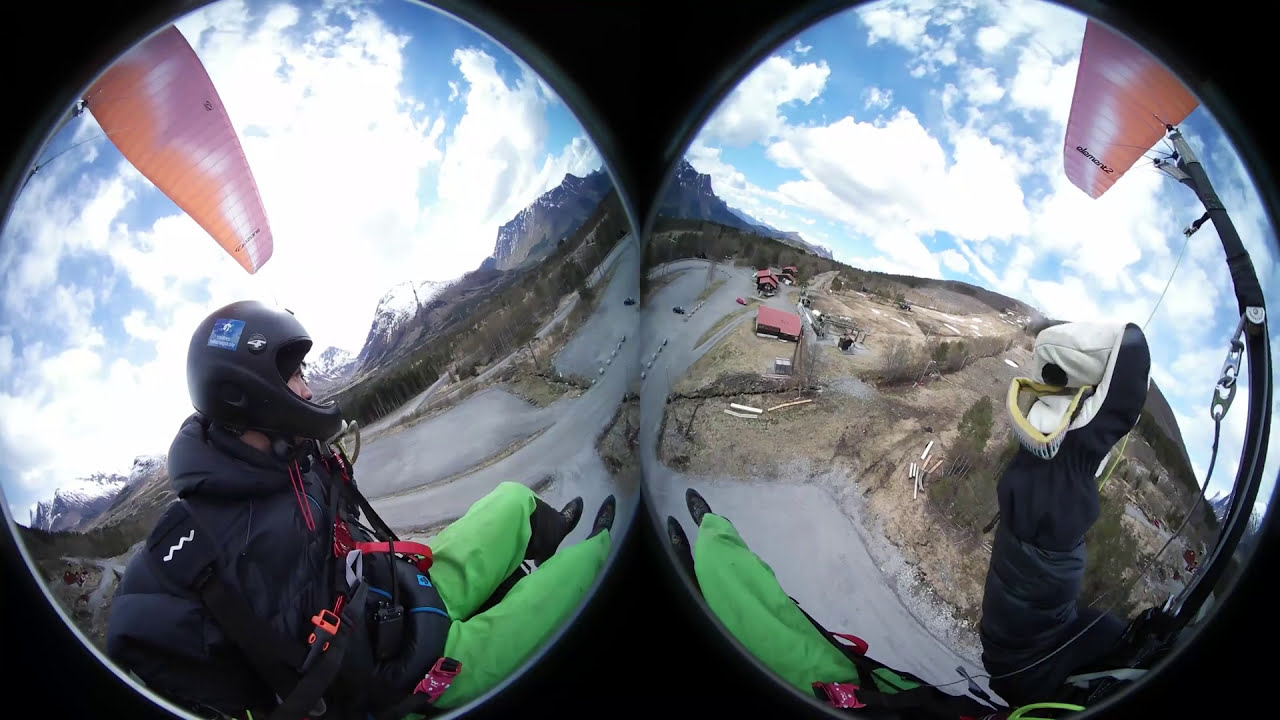The image presents a split-view scene through two fisheye telescope lenses depicting the same person from different angles, as if mirrored. On the left lens, a woman is sitting atop a mountain or hill, donning a black helmet, black jacket, green pants, and black shoes. She appears poised for paragliding, evidenced by the presence of a red wing overhead connected via a cable apparatus. On the right lens, only her right arm and two legs are visible, again showcasing the same black jacket, green pants, and black shoes, with her hand clutching a small white bag. The background features a mountainous landscape with a path leading up to the snow-capped peaks. The sky is a vivid blue, dotted with heavy white clouds, and the ground below shows sparse buildings and lumber, indicative of a high-altitude launch point above the tree line. The overall scene suggests a moment of anticipation before a paragliding adventure.